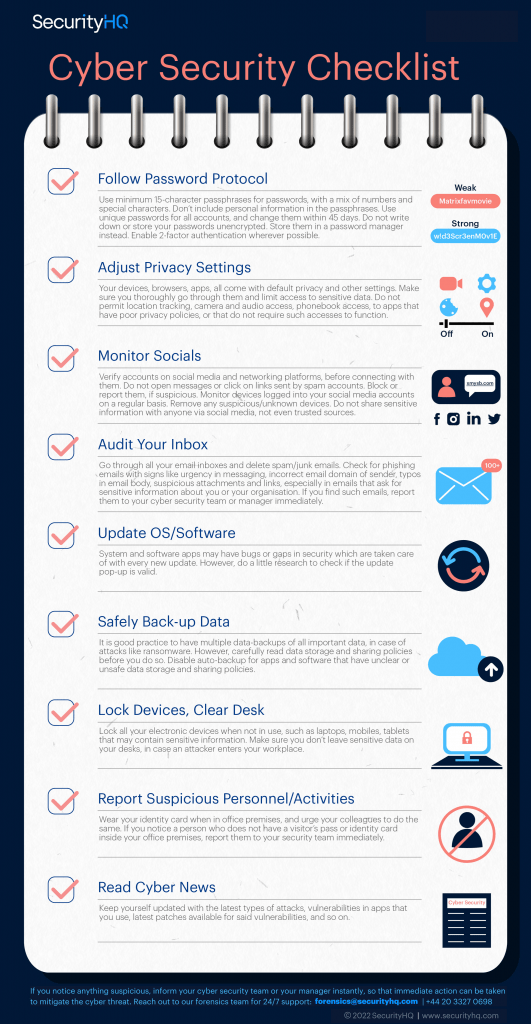The image features a dark navy blue background with a Cyber Security Checklist prominently displayed at the center, designed to resemble a spiral notebook. At the top, the words "Security HQ" are written in white and blue letters, while "Cyber Security Checklist" is highlighted in red letters against the dark backdrop. The checklist consists of ten essential tasks, each accompanied by colorful illustrations to represent the activities:

1. **Follow Password Protocol** – Ensuring strong, unique passwords.
2. **Adjust Privacy Settings** – Customizing privacy configurations.
3. **Monitor Socials** – Watching for unusual activity on social media.
4. **Audit Your Inbox** – Checking emails for security threats.
5. **Update OS Software** – Keeping operating systems current with updates.
6. **Safely Backup Data** – Represented by a cloud with an upward arrow, highlighting the importance of data backups.
7. **Lock Devices** – Securing all devices with locks.
8. **Clear Desk** – Maintaining a clutter-free workspace to prevent security breaches.
9. **Report Suspicious Personnel/Activities** – Vigilantly reporting anything unusual.
10. **Read Cyber News** – Staying informed about the latest in cyber security.

To the right of each item, small graphics provide visual cues—such as an envelope icon for auditing your inbox or a cloud for backing up data—while checkboxes to the left indicate completion. Each item includes brief definitions, though they are blurry and difficult to read. At the bottom of the page, there appears to be additional text, likely disclaimers or contact information, but it’s also blurry and unreadable.